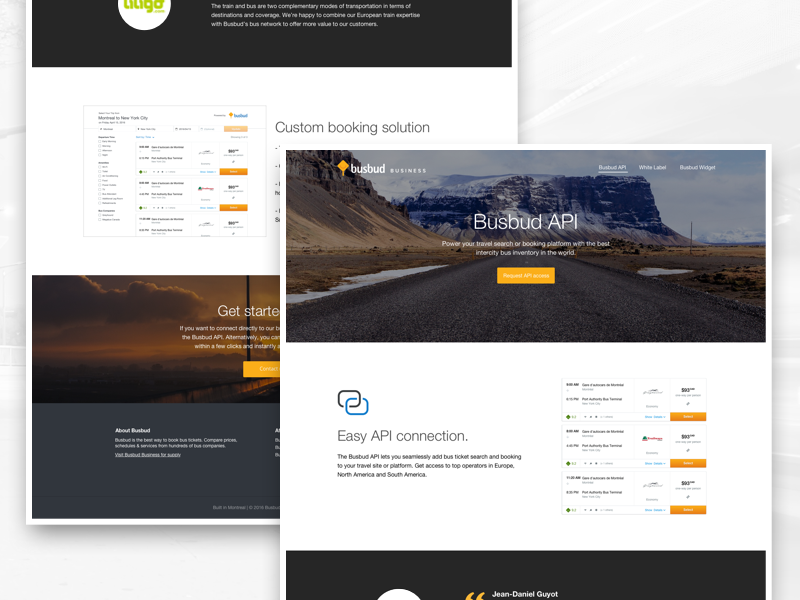The image features a slightly wider than tall layout showcasing two overlapping website interfaces. The first website originates from the upper left of the image, occupying about 80% of the height and two-thirds of the width. It features a header positioned approximately a third of the way down its right half, displaying the text "Custom Booking Solution." The left side of this website is faintly visible, revealing a few orange clickable buttons accompanied by some indistinct text. The bottom part of the page is dominated by a banner depicting a cloudy scene cloaked in a brownish haze, with the phrase "Getting Started" prominently displayed and an orange button beneath it.

The second website starts roughly a third down from the top and a third over from the left side, overlapping the bottom right section of the first website. It showcases an image of a road leading towards distant mountains with the text "Busbud API" positioned at the center. Below this, there’s the phrase "Easy API Connection" set against a white background. The right side of this section includes additional orange buttons and text.

Overall, the dual-layered webpage presentation is intricately detailed yet small in size, making individual elements tough to discern clearly.